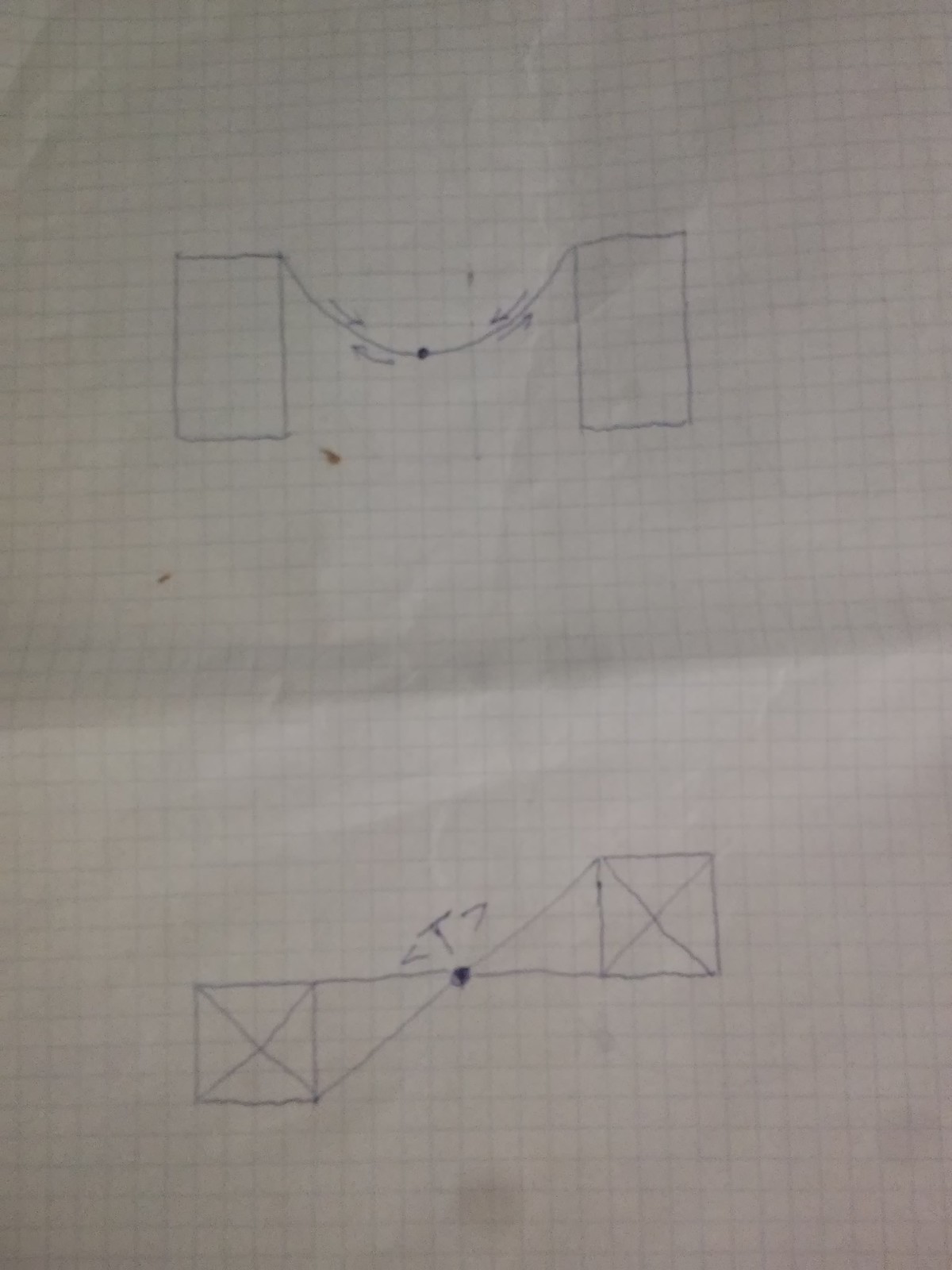This image displays two intricate schematic drawings on a slightly creased, lined white paper. The lines on the paper form a grid of elongated rectangles rather than squares. 

The top drawing features two squares connected by a gently curved, U-shaped line. There is a prominent dot in the center of this U-shape, with arrows pointing towards it from the squares and also towards the squares from the dot.

The bottom drawing also begins with two squares, but in this illustration, the squares are staggered rather than aligned side by side. Each square has an X marked through it. Instead of a U-shaped connection, the squares are linked by an hourglass shape. Similar to the first drawing, there is a central filled dot here as well. Additionally, this drawing includes a T shape with two sideways V's positioned nearby.

The meticulous detailing of the drawings suggests a conceptual or possibly technical design, conveyed thoughtfully with arrows and symbols to illustrate the relationships between the elements.